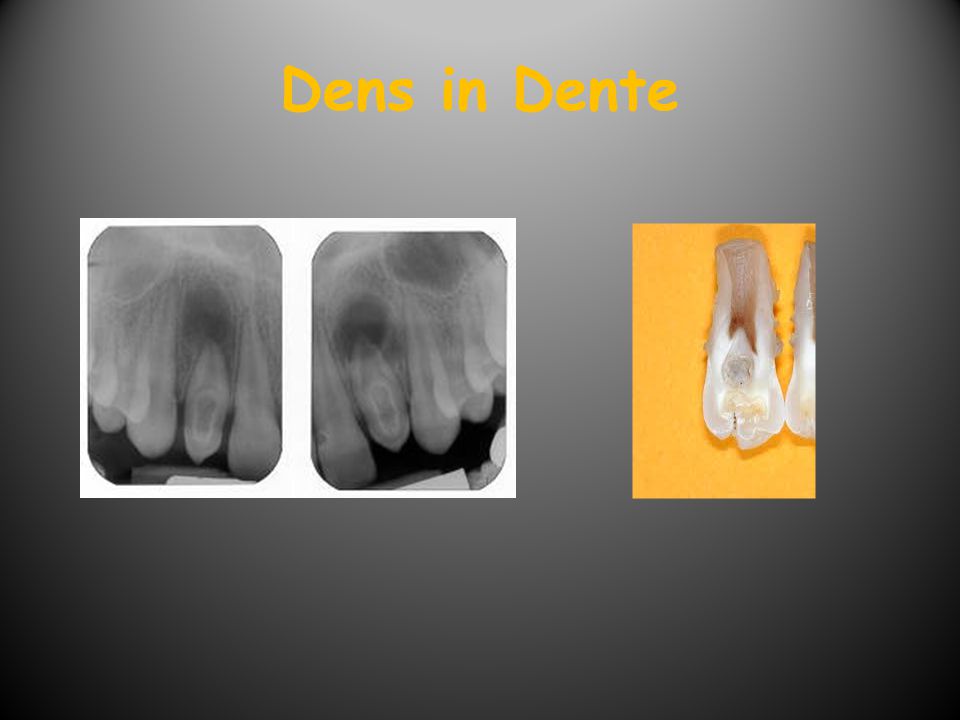The slide titled "Dens in Dente" features a gray background that gradients slightly darker towards the edges. Written in yellow, centered at the top, is the title "Dens in Dente," with "D-E-N-S" and "D-E-N-T-E" in capital letters, and "in" in lowercase letters. Below the title, three images of teeth are presented. On the left side, within a white rectangle, are two black-and-white dental x-rays, each showing teeth with notable structural anomalies. To the right, there is a color photograph of an extracted tooth, partially showing another tooth, set against a yellow background. The base slide adds depth through its color gradient, and the layout draws a clear comparison between x-ray observations and real-life dental extractions.